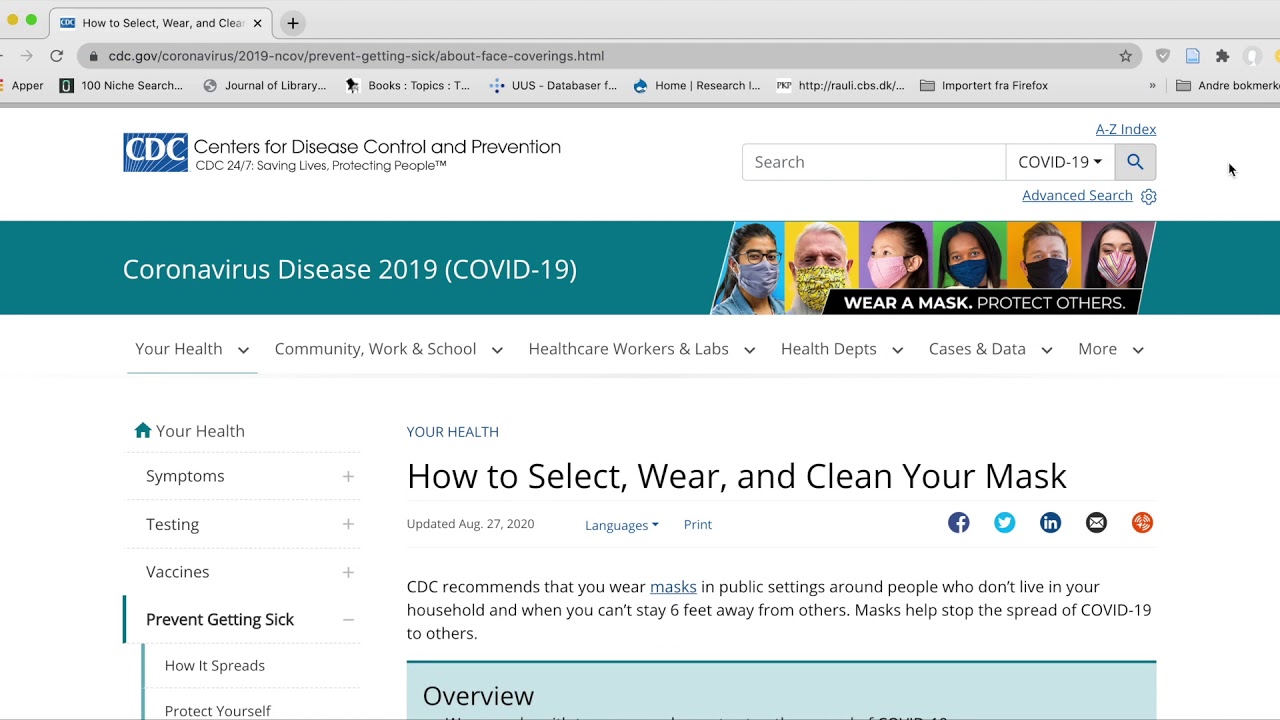The image is a screenshot of a specific section of the Centers for Disease Control and Prevention (CDC) website, focusing on guidance related to the coronavirus disease 2019 (COVID-19). The section highlighted is titled "Prevent Getting Sick" and provides detailed information on mask usage. Published on August 27, 2020, the CDC advises wearing masks in public settings, especially where maintaining a six-foot distance from others is not feasible, to help curtail the spread of COVID-19. The page elaborates on how to select, wear, and clean masks. Above this section, there is an image depicting six individuals, each wearing different styles of custom face masks, accompanied by a banner that reads, "Wear a mask, protect others." The overall tone underscores the critical public health message of mask-wearing to protect the community.